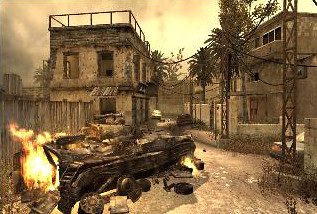The image depicts a loading screen for a Call of Duty map, designed with a detailed, post-apocalyptic ambiance reminiscent of the 2000s era of the game franchise. Central to the scene is a destroyed, burning tank in the left middle ground, emitting flames and enveloped in thick, black smoke. Nearby, there is a car, also damaged, hinting at extensive vehicular destruction. The setting appears to be a tropical, yet deserted town, characterized by a light tan hue that blankets the image.

Flanking the tank are remnants of permanent structures; there is a burnt-out shell of a building situated in the back left corner, contributing to the war-torn atmosphere. A large wooden fence lines part of the area, while broken power lines and metal beams add to the scene’s desolation. 

In the background, you can discern tall palm trees standing amidst the devastation, and a variety of clouds — from light to dark gray — casting a gloomy shadow over the environment. The ground is predominantly brown, conveying a dry, dusty texture. The overall environment is foggy and hazy, further contributing to the abandoned and chaotic feel of the town.